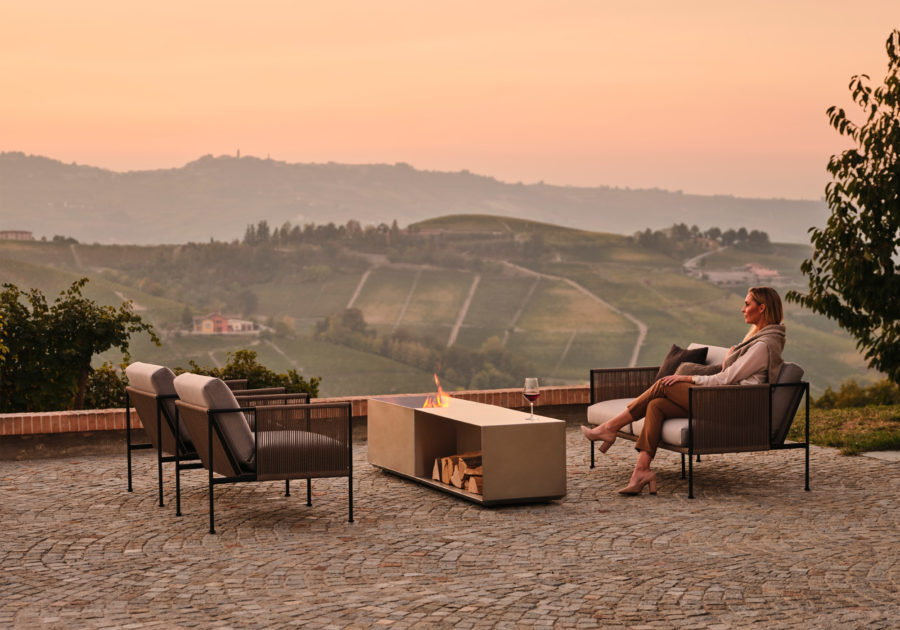In this serene and picturesque photograph, a woman is sitting on a beige cushioned sofa with a black frame, part of an elegant outdoor patio setup. She’s dressed in beige tones including brown pants, high-heeled beige shoes, and a beige top with a matching scarf or sweater draped around her neck. With her dirty blonde hair gently catching the light, she sits with her legs crossed, gazing into the distance, exuding relaxation and poise. The patio features a brick surface of brown and gray stones, harmonizing with the comfortable outdoor furniture. To her left, two black lounge chairs with beige cushions mirror her sofa’s color scheme and flank a unique coffee table integrated with a fire pit adorned with burning logs. A partially filled wine glass rests on this table, adding to the tranquil ambiance.

The backdrop is a breathtaking vista of rolling green hills dotted with farms and houses, framed by a pink-orange misty sunset sky. Far off in the distance, the horizon is softened by foggy mountains, contributing to the image's serene and elegant feel. A green bush is visible to the left of the patio, while a tree stands tall to the right, adding to the lush environment. The overall composition captures a perfect blend of nature's beauty and sophisticated outdoor living.